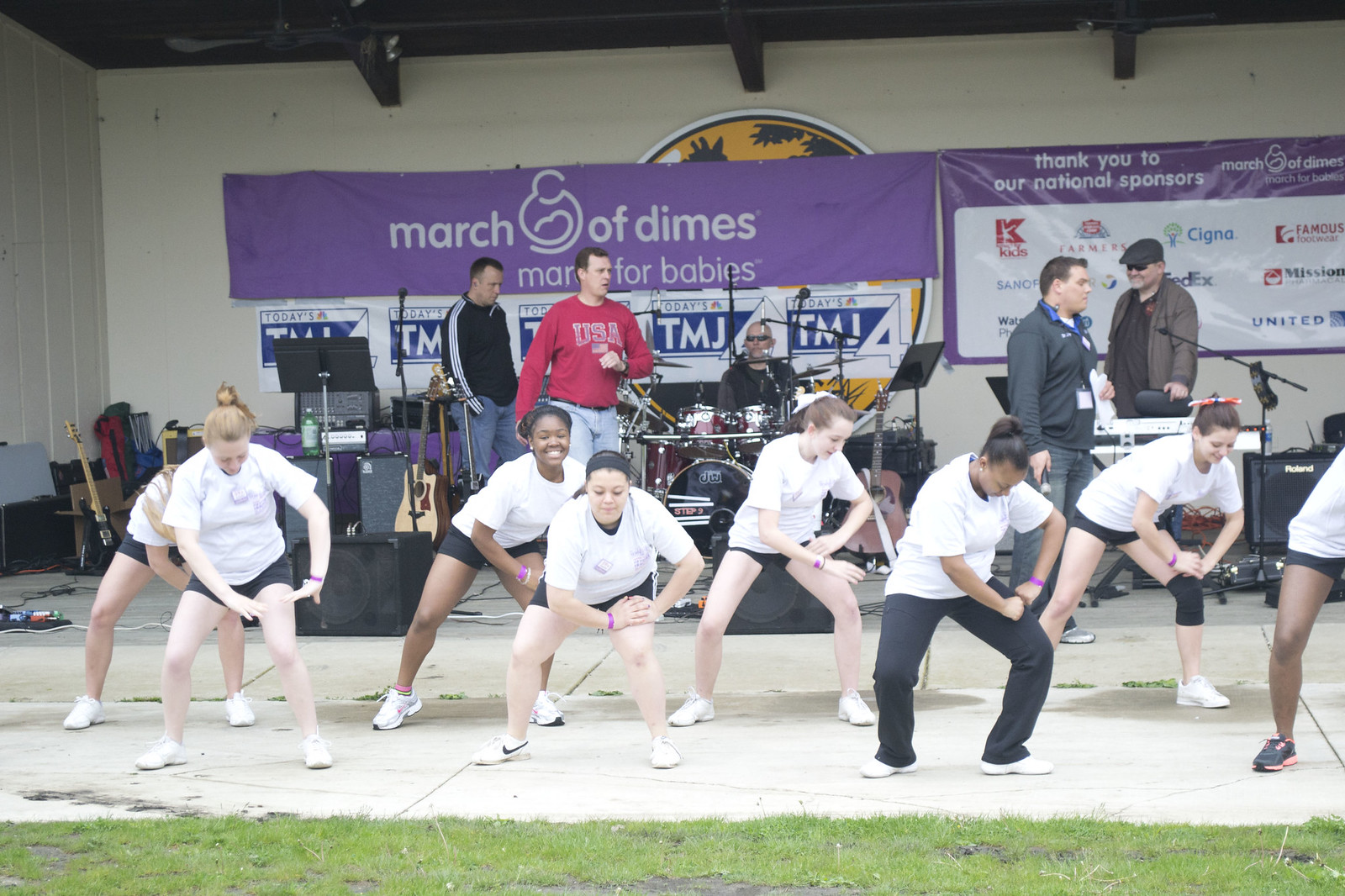This horizontally aligned rectangular image captures a vibrant moment at a charitable event, likely outdoors during the day. In the foreground, eight young women, including three black and five white individuals, are performing a dance - seemingly the "stanky leg" - on a sidewalk area with some grass visible at the very bottom of the picture. They are all clad in white t-shirts and black shorts, except for one in front wearing black pants. The dancers have their hands on their left legs, with knees bent and leaning down, and they are smiling for the camera, embodying a joyful spirit.

Behind them stands a wall adorned with purple and white banners. The prominent banner reads "March of Dimes, March for Babies," along with a thank you note to national sponsors featuring logos from companies like United, Cigna, FedEx, Famous Footwear, Farmers Insurance, and the NBC network, among others. Additionally, five men are seen in the background next to musical equipment; one is seated at the drums while the others stand, with notable attire including a red long sleeve shirt with "USA" on it and a black and white striped long sleeve top.

This colorful and detailed scene captures the essence of community and support, encapsulating the spirit of the event and its participants.